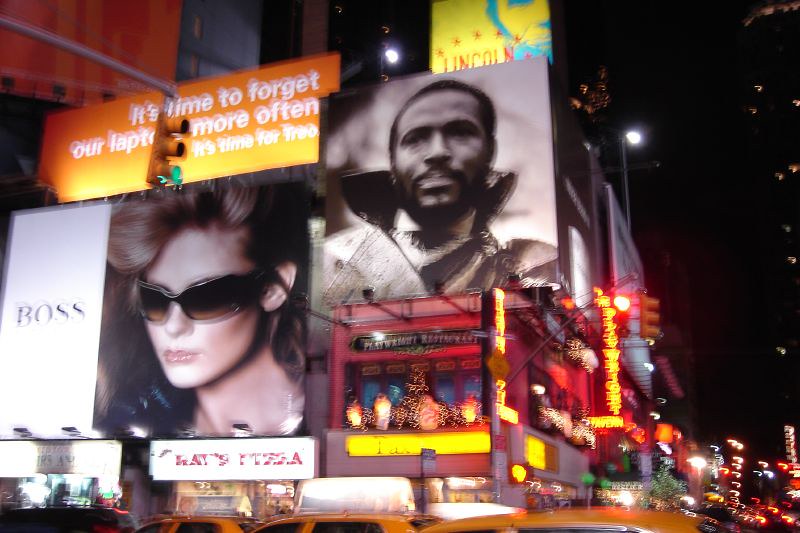A nighttime photograph of Times Square, New York City, brimming with the iconic vibrancy and energy of the location. The image is somewhat blurry, adding a layer of mystique to the bustling scene. Dominating the center and bottom right is Ray's Pizza, a well-known New York landmark. Above, an array of illuminated billboards captures the eye: a conspicuous orange billboard just behind a green traffic light reads, though somewhat indistinctly, "It's time to forget our laptops more often. It's time for travel, maybe?" A bright yellow billboard prominently features Abraham Lincoln's face in blue and the word "Lincoln" in red, surrounded by stars. Below Lincoln's billboard, a black and white image of Marvin Gaye is displayed. Adjacent to the orange billboard is an advertisement for Boss, adding to the commercial tapestry of lights and messages.

Further to the right is a red sign for the Playwright Restaurant, partially visible through a large window illuminated by internal lights. Below it, a yellow neon sign adds to the vivid atmosphere, though its text is obscured. The building turns a corner further along the street, showing another yellow sign and a descending red neon sign, while a traffic light glows red at this intersection.

The photograph's middle and foreground are speckled with the indistinct tops of cars or taxis, hinting at the ceaseless flow of traffic typical of Times Square. Towering above, tall buildings frame the scene, their silhouettes punctuated with countless twinkling lights, embodying the essence of New York City’s nightlife.